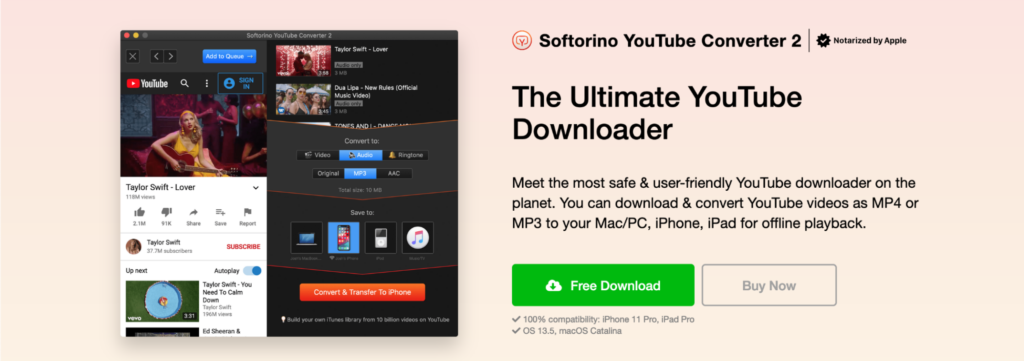In this image, a prominent pink box dominates the layout. On the left side, there is a black screen featuring a small, red YouTube logo. The screen displays various icons and pictures, including an image of a girl, a film clip, and a couple of blue buttons. Additionally, there's a blue square and a circle with music notes alongside a red button. An inset on the screen displays the name "Taylor Swift" and the title "Lover", indicating that users can listen to the song.

On the right side of the image, there is a red circle with another circle inside it, containing a small red heart. This section highlights the "Softorino YouTube Converter 2" and includes a black circle with a check mark, accompanied by the message "notarized by Apple." The text hails this as "the ultimate YouTube downloader" and promotes it as being safe and user-friendly. It mentions that the software allows users to download and convert YouTube videos to mp4 or mp3 formats on their Mac, PC, iPhone, or iPad for offline playback.

Below this section, a green button with a white cloud and a green downward arrow offers a "Free Download" option, while a pink button outlined in blue provides a "Buy Now" option in light blue text. The image also includes two check marks indicating 100% compatibility with the iPhone 11 Pro, iPad Pro, and OS 13.5.